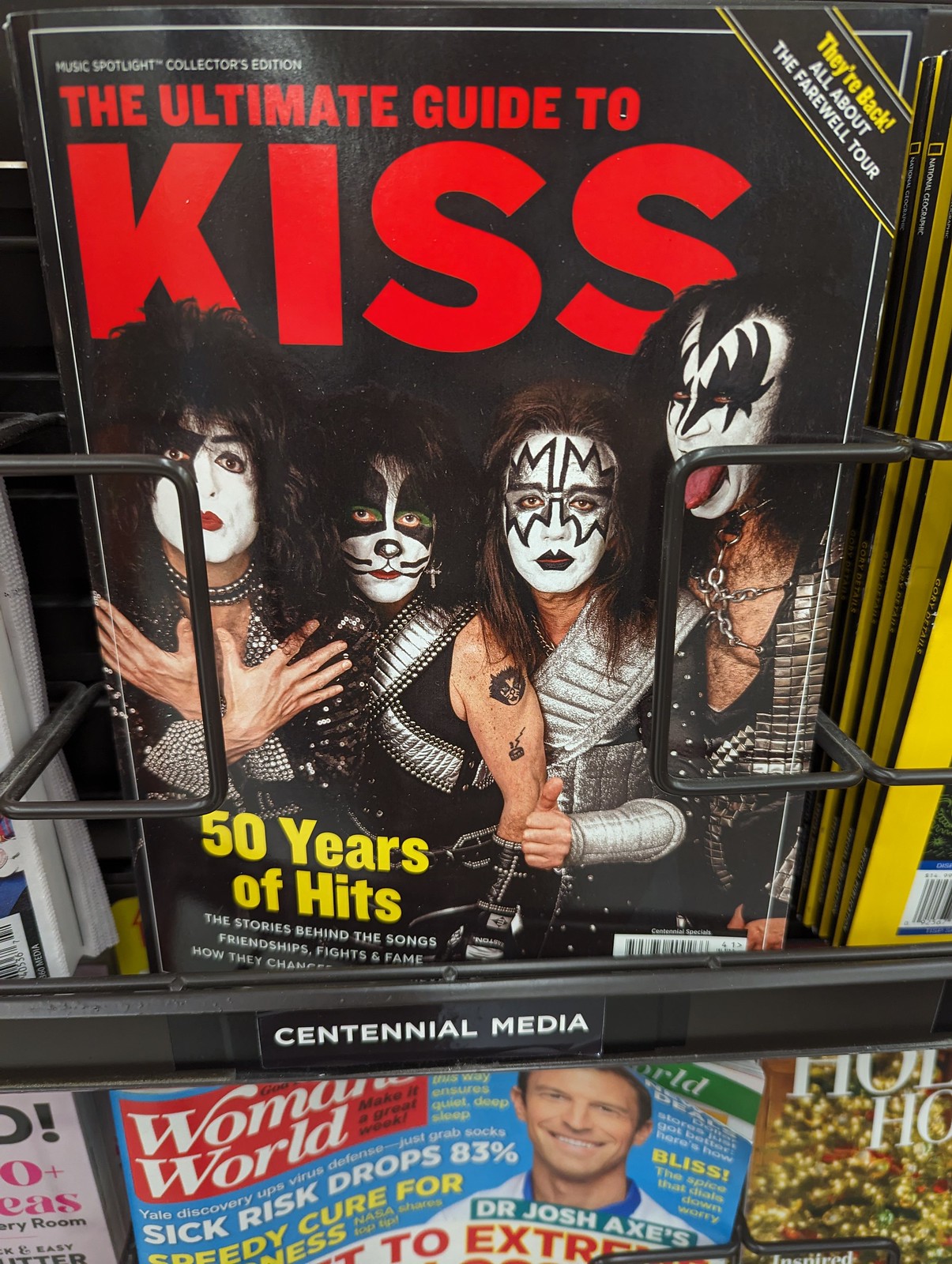The image is a close-up of a magazine rack typically found near the checkout at a grocery store. The focal point of the photograph is a magazine with a prominent black cover titled, "Music Spotlight Collector's Edition, The Ultimate Guide to Kiss," with the subtitle in red. A diagonal yellow stripe on the right corner boldly announces, "They're Back," with "All About the Farewell Tour" written in white beneath it. The central photograph features the four iconic members of the band Kiss, each with their signature black and white face makeup and long black hair. They are dressed in striking black and silver outfits, with one member giving a thumbs up and another striking a pose with arms out like a butterfly. The bottom of the cover reads, "50 Years of Hits," in yellow, followed by "The stories behind the songs, Friendship, Fights, and Fame," in white. The magazine is displayed on a rack labeled Centennial Media, and the top of another magazine titled Women’s World is visible below it.